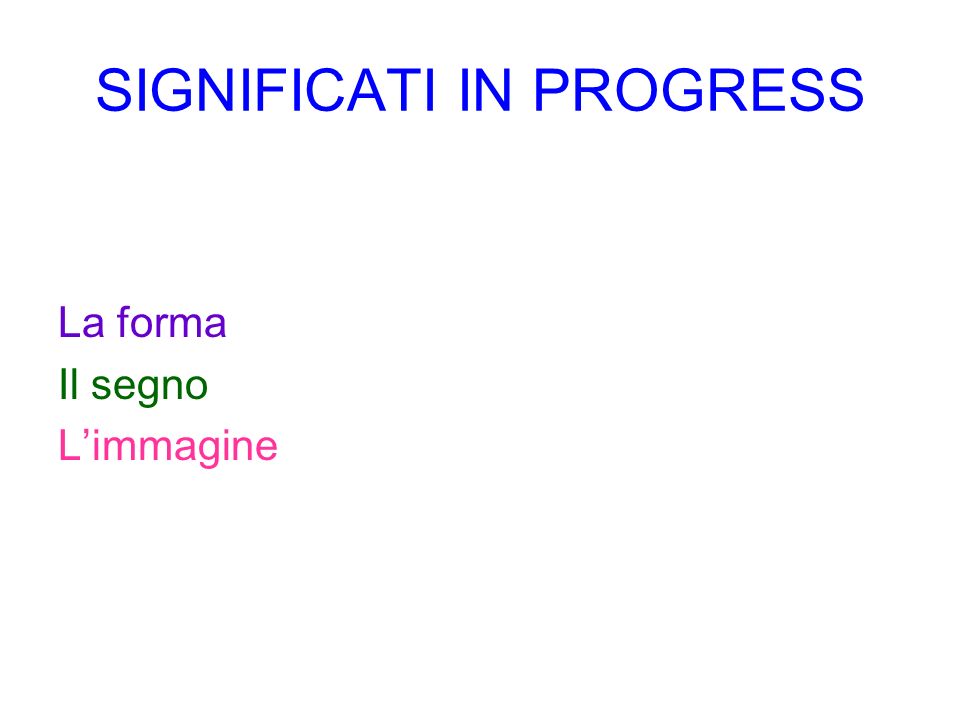The image features a horizontal rectangle with a white background displaying colored text. At the top center, in large blue capital letters, it reads "SIGNIFICATI IN PROGRESS." On the bottom left, there are three lines of smaller text, each in a different color. The first line, in purple, says "La Forma" with the 'L' capitalized. Directly below it, in green text, it reads "Il Segno." The final line, in pink, states "L'Immagine" with a capital 'L.' The font throughout the image is a regular, non-script style, resembling Helvetica. This layout, with its minimalistic design and colored text on a plain white background, suggests it could be an internet sign, flyer, or a website headline.